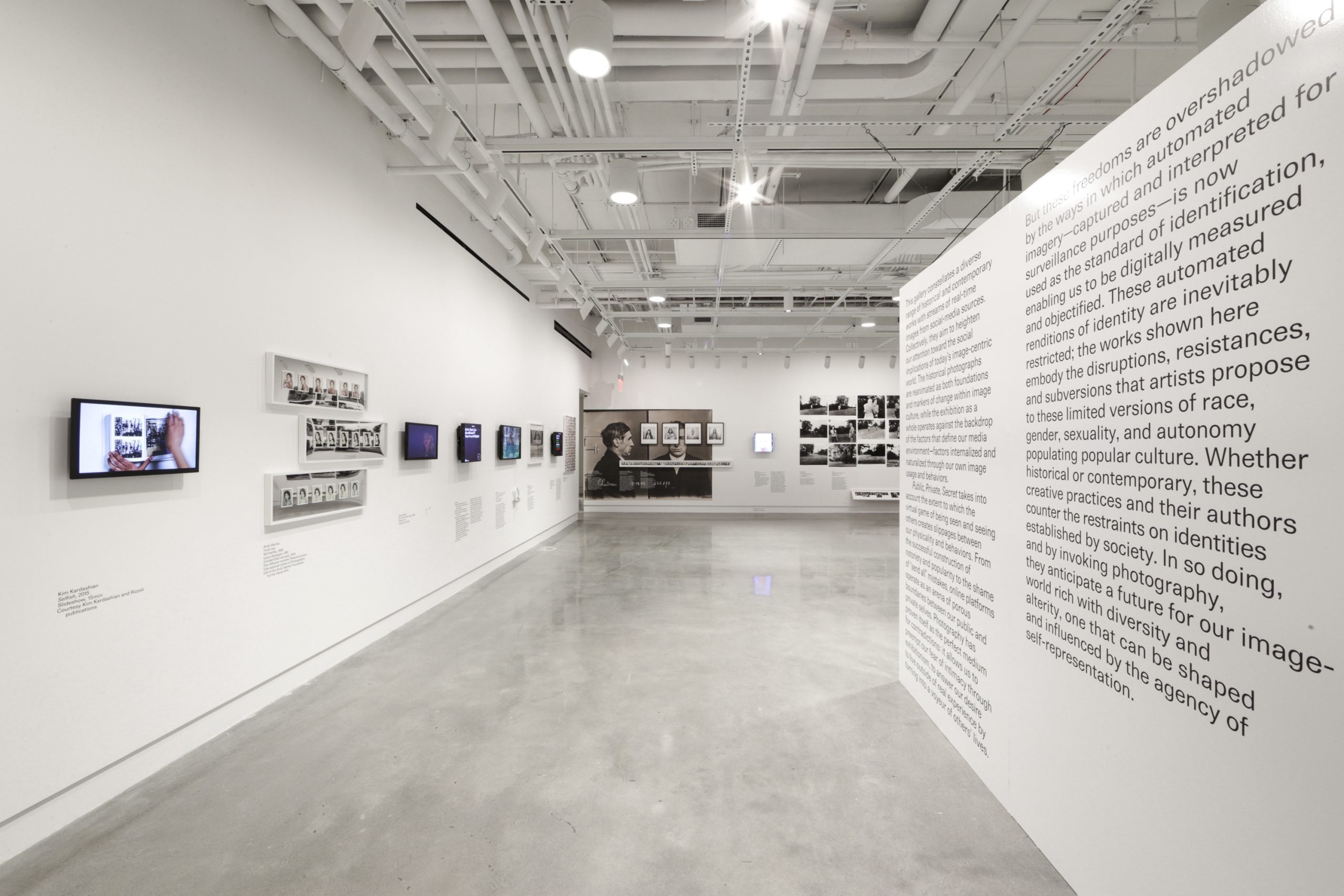The image depicts a long hallway in a spacious, high-ceilinged office or exhibit space with an open, industrial aesthetic marked by exposed pipes and bright lights. The floors are sleek and gray, likely polished concrete. The walls are a sterile white, contributing to the stark, monochromatic ambiance of the room. The right wall is densely covered with extensive black text, possibly in a typewriter font, discussing themes such as culture, autonomy, and disruption. The left wall features numerous digital displays and photographs, some resembling small, colorful monitors or digital picture frames. Towards the back of the hallway, a large black-and-white photograph is prominently visible. The overall effect is a blend of modern technology and minimalist design, suggesting it could be a marketing or tech office, or even a contemporary art exhibit.